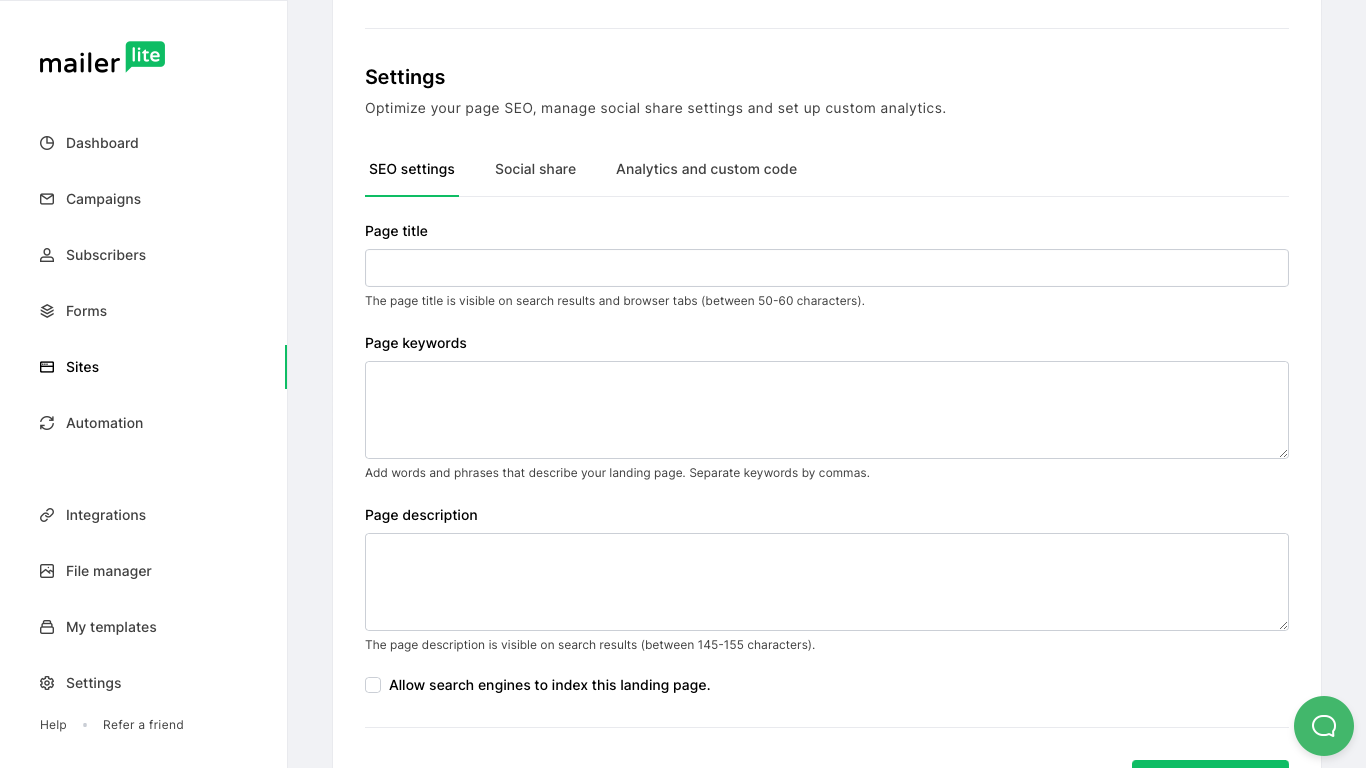The image depicts the "Settings" page within the Mailer Lite web application, which is apparent from the left-hand navigation menu and the detailed settings panel.

On the left-hand side, there's a vertically-aligned navigation menu set against a white background. At the top of this menu, the Mailer Lite logo is displayed, with the word "Mailer" in black lowercase letters, followed by the word "Lite" in white lowercase letters inside a green box. Below this, there is a list of menu options:

1. **Dashboard** - Represented by a circle icon.
2. **Campaigns** - Indicated by an envelope icon.
3. **Subscribers** - Illustrated with a silhouette icon.
4. **Forms** - Shown with a stack of papers icon.
5. **Sites** - Depicted with a square icon.
6. **Automation** - Highlighted with two arrows forming a circle icon.
7. **Integrations** - Symbolized by two chain links icon.
8. **File Manager** - Shown with a square icon.
9. **My Templates** - Represented by a briefcase icon.
10. **Settings** - Iconified with a gear.

At the bottom of this menu, the options "Help" and "Refer a Friend" are listed.

The central part of the screen is the "Settings" page, bordered on both sides by vertical gray lines, which segment this area from the menu on the left and any additional content to its right. The background of the settings panel is also white. At the top, the page prominently displays the title "Settings," followed by a brief description: "Optimize your page SEO, manage social share settings, and set up custom analytics."

Below this header, there are three selectable sections—"SEO Settings," "Social Share Analytics," and "Custom Code." Currently, the "SEO Settings" section is active, distinguishing itself with a green underline.

Within the active "SEO Settings" section, there are several fields and instructions:

1. **Page Title** - An input box for the page title, with a guideline below stating, "The page title is visible on search results and browser tabs (between 50 to 60 characters)."
2. **Page Keywords** - A blank input box for keywords, accompanied by the message, "Add words and phrases to describe your landing page. Separate keywords by commas."
3. **Page Description** - Another input box, with the note below reading, "The page description is visible on search results (between 14 to 155 characters)."
4. **Allow Search Engines to Index This Landing Page** - A checkbox that remains unmarked.

At the bottom-left corner of the settings panel, there's the top portion of a green square visible, with a round green circle to its right containing a white speech bubble, possibly serving as an icon for further options or help.